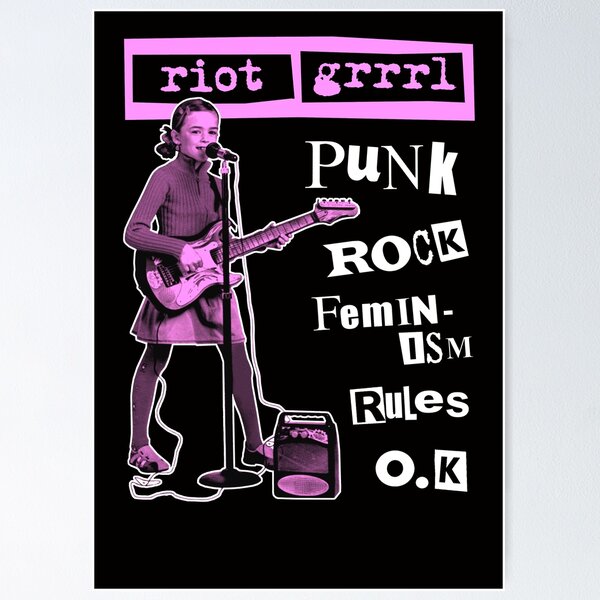This event poster, predominantly black, vividly features a bold design with scrapbook elements. The top section contains a prominent pink rectangle with smaller black squares and bold pink text that reads "Riot Grrrl" (spelled G-R-R-R-L). Below it, a young girl is depicted standing and playing a bass guitar while singing into a microphone. The guitar cord connects to a microphone stand, and another wire leads to an amplifier near her right foot. She is adorned with short, shoulder-length hair styled in double ponytails tied with bows, a long-sleeve shirt, a skirt, leggings, and small shoes. Her outline is tinted pink, accented with black and brown patches. To her right, between the head and neck of the guitar, are white cut-out letters spelling "punk," followed by "rock," "femin-," and "ism," ending with "rules OK," arranged in a stylized, ransom note-like fashion. The overall aesthetic gives a playful, DIY scrapbook-like vibe that emphasizes themes of punk rock and feminism, embodied in the energetic image of the young, performing girl.